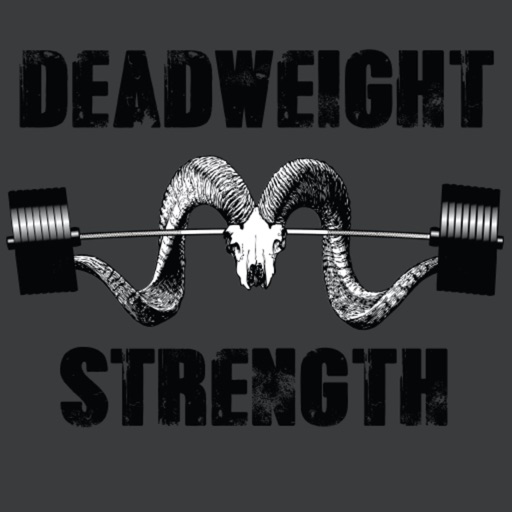The poster resembles a gym advertisement, featuring a striking black and white color scheme. Central to the design is the skull of a ram, its curved horns wrapping around a heavily loaded barbell that bends under the weight. The entire image is set against a dark gray background. At the top of the poster, "DEADWEIGHT" is written in a scuffed, weathered black font, while at the bottom, “STRENGTH” appears in the same distressed style. The text appears to be stenciled on, giving the entire composition a rugged, worn-out look that matches the overall aesthetic. The clear focal point is the ram's skull and barbell, whereas the background and text seem faded and distressed, reinforcing the gritty, intense vibe characteristic of a challenging gym environment.